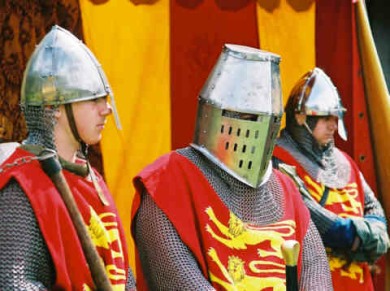The photograph captures a scene reminiscent of a medieval or renaissance festival, featuring three men dressed in knightly battle armor. Each man is adorned in iron or steel helmets, with two showing their faces and the top of their heads covered, while the man in the middle is wearing a full-face helmet. They are clothed in iron chainmail with red surcoats bearing a crest with three yellow lions. One man casually holds a spiked mace over his shoulder, though the weapon is partially out of view. In the background stands a tent with alternating red and yellow stripes, suggesting a campsite or staging area for the event. The men appear ready for action, possibly preparing for a reenactment or mock battle at a renaissance fair.